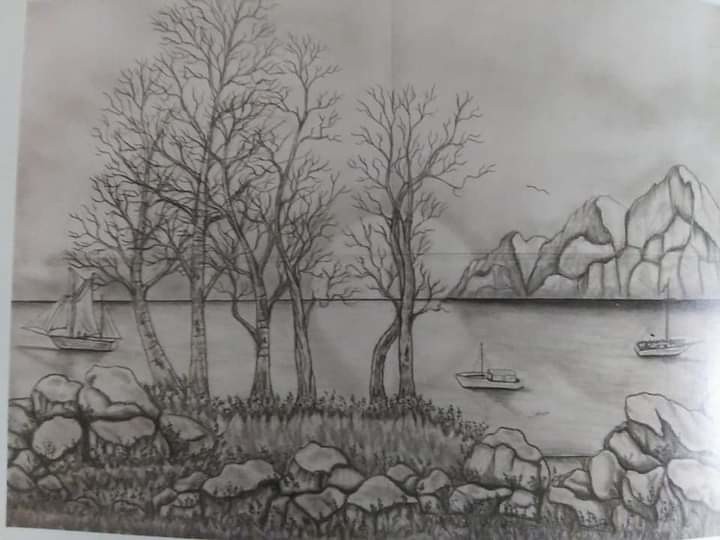This detailed black-and-white pencil drawing, rendered on a white piece of paper, captures a serene, natural landscape. In the foreground, a grassy shore is scattered with various-sized rocks, ranging up to boulder size, and is interspersed with leafless tree trunks hinting at a wintry scene. Further down the shore, there's sparse vegetation, including patches of grass and brush. Beyond the shore lies a calm body of water, reflecting the gentle stillness of the scene. Three boats traverse the water; to the left, a sailboat with three large sails gracefully heads towards the left, while on the right are two smaller boats, possibly fishing vessels, with their sails not unfurled. Stretching across the background is a rocky, maybe even mountainous, terrain, devoid of vegetation and suggesting either a rugged landscape or snow-covered peaks. Above this tranquil tableau, a single bird is silhouetted against the cloudy sky, adding a touch of life to the otherwise still scene.